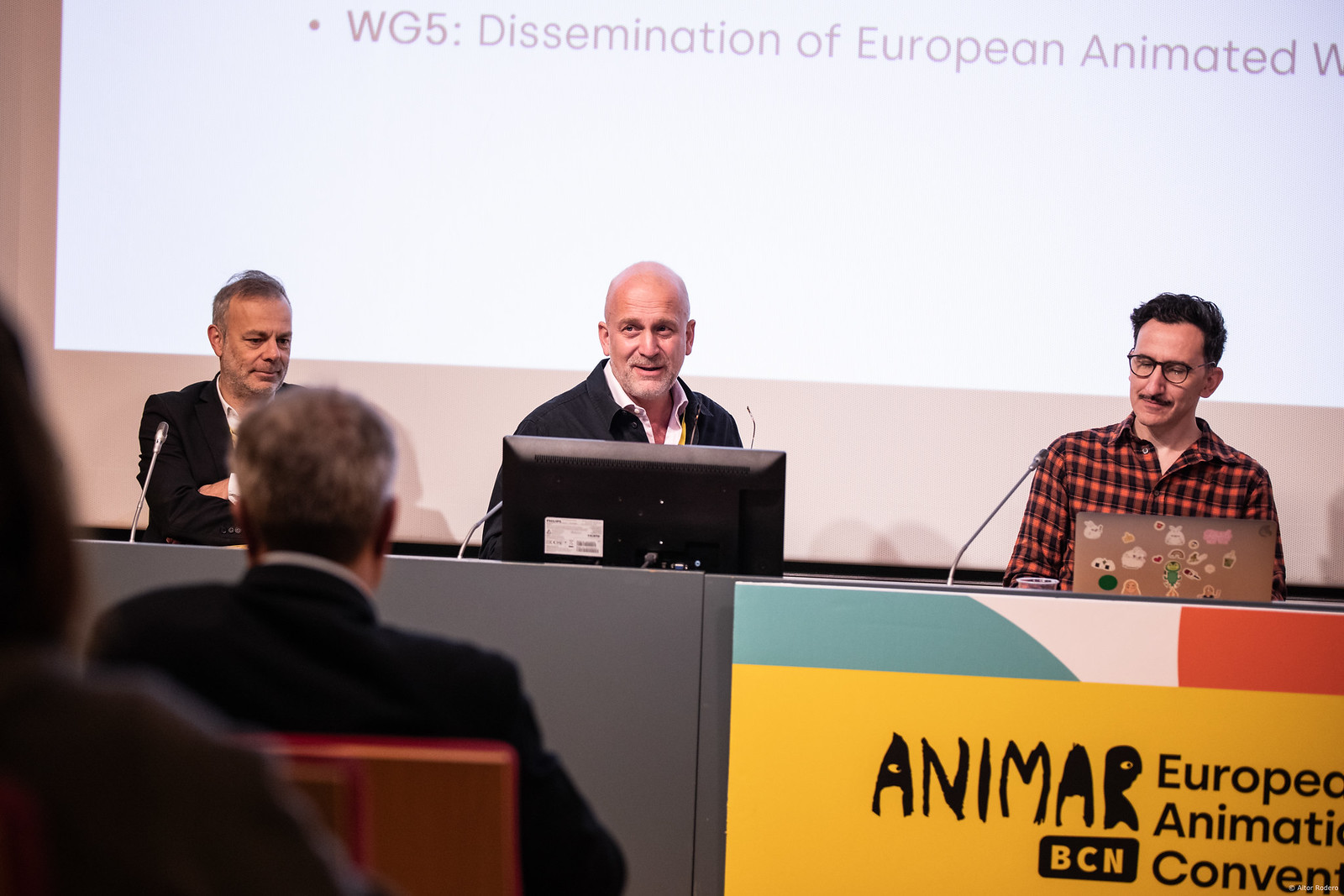This photograph captures a panel discussion at what appears to be a European animation convention, likely inside a convention center or meeting hall. The focus is on three men positioned horizontally in the center of the image, each sitting in front of a microphone. Behind them, a white projection screen partially displays the text "WG5 Dissemination of European Animated," along with some other cut-off text. 

The man on the left is dressed in a black suit jacket and is sitting with his arms crossed, smiling while looking down. The central figure stands behind a desktop computer, dressed in a dark jacket with a button-up shirt underneath and a lanyard around his neck, smiling at the audience. On the right, a man wearing a plaid orange and black shirt, glasses, and a mustache sits in front of a laptop decorated with stickers. 

In front of the panel, a sign prominently features the word "Animar." The backdrop includes additional signage in yellow, light blue, orange, and white colors with black text, hinting at the context of a European Animation Convention in Barcelona (BCN). The bottom portion of the image shows the silhouettes of two audience members, with the back of one man in a dark jacket and gray hair clearly visible, suggesting they are engaged and watching the presenters.